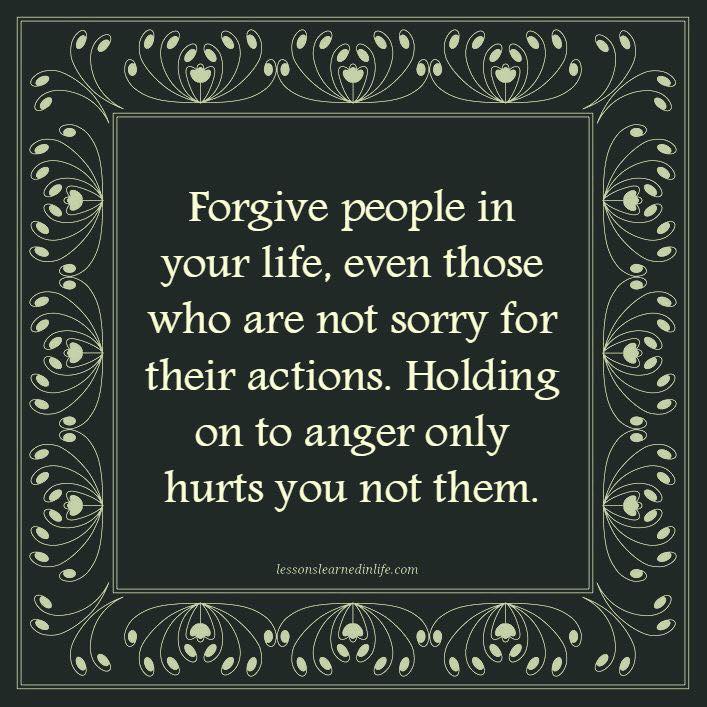The image is a digitally generated inspirational quote with a decorative design. It features a central black square with a light green or off-white inscription that reads, "Forgive people in your life, even those who are not sorry for their actions. Holding on to anger only hurts you, not them." This quote is centered within the black square. Surrounding this central square is another square with a dark green border, adorned with graphics resembling lily flowers and stems, giving it the appearance of a framed picture. Below the quote, within the black square, the website "lessonslearnedinlife.com" is displayed, providing the source of this motivational message.